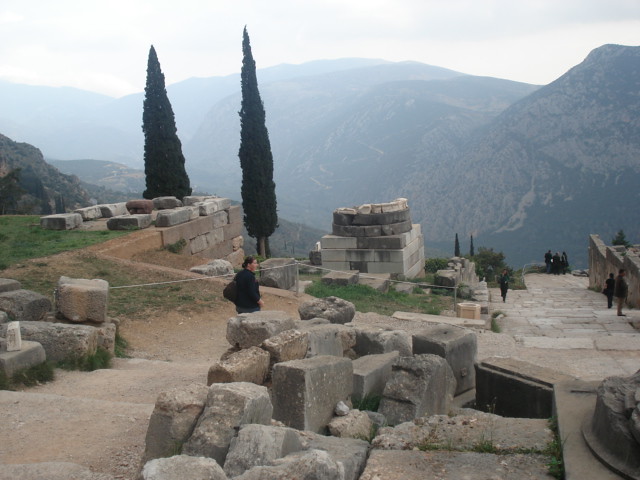This outdoor photograph captures the edge of a cliff that has been carefully landscaped, suggesting the presence of ancient ruins or a historic site. Prominent in the foreground are stone walls and large steps forming a manicured walkway flanked by boulders that have been intentionally placed. A single person, dressed in black, is walking down the steps with a few others further below to the right, more distant. To the left, there are carefully pruned cedar trees adding a touch of greenery.

The walkway features a rope handrail for safety and appears to guide visitors along the cliffside, possibly serving as a sightseeing spot or overlook. Below the cliff, one can infer a valley stretching out, with rugged mountains rising majestically in the background. The sky above these mountains is overcast, contributing to the photograph’s somewhat dull and misty ambiance. The image, likely slightly overexposed at the top, reveals the natural beauty and historical significance of this tranquil, yet awe-inspiring location.